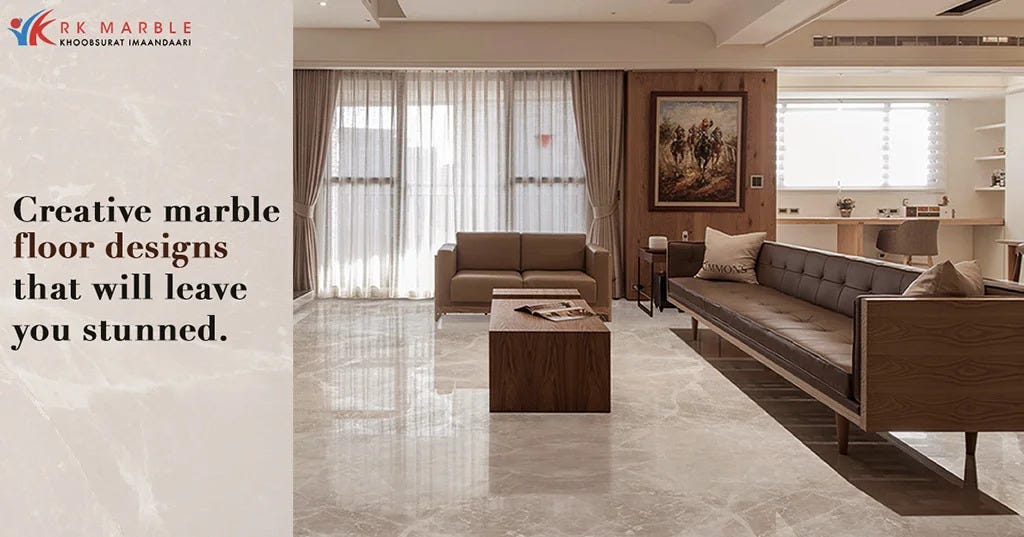This advertisement for RK Marble features an elegantly decorated living room showcasing the company’s stunning marble flooring. The white-gray, ivory-toned marble floor is highly polished, with streaks and whorls that beautifully reflect the room's furnishings. The room includes a lengthy brown leather couch and a matching small loveseat, both adorned with beige pillows. A wooden coffee table holds an open magazine, adding a touch of lived-in sophistication.

To the left, a large sliding glass door draped with white and beige curtains suggests an attached deck, allowing plenty of daylight to flood the space. On the right, a wooden desk is positioned next to a window equipped with white blinds, adding a functional workspace to the serene living room. In the center of the room, a striking painting of people riding horses adds a touch of artful elegance, and beneath it, a modest air purifier and a thermostat further enhance the room's modern comforts.

The ad’s text, displayed in a mix of black and brown, reads: “Creative Marble Floor Designs That Will Leave You Stunned,” underscoring the luxurious appeal of their product. At the top of the image, RK Marble’s logo proudly sits, promising exquisite design that transforms any space. The overall color palette of light brown and beige creates a calming and welcoming atmosphere, perfectly complementing the lustrous marble floor.